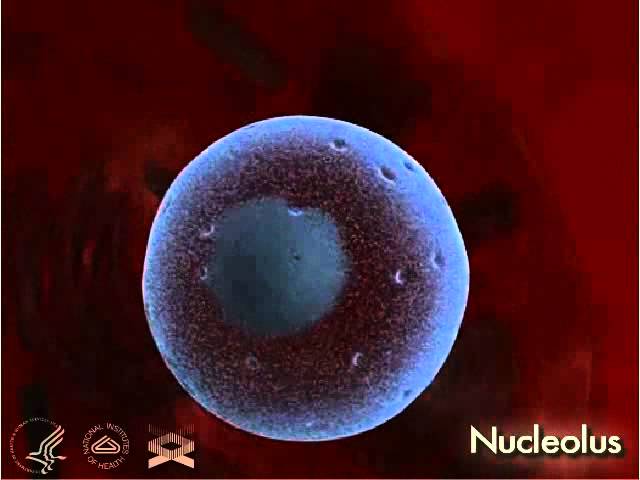The image depicts a highly pixelated, low-resolution representation resembling a nucleolus, prominently labeled in the bottom right corner with white, yellowish letters reading "NUCLEOLUS." This centrally glowing, gradient blue circle features darker, porous patterns towards its center, transitioning to a greenish-blue hue, mimicking organic cellular structures. The circle is set against a deeply red, gradient background, evoking an organic, almost blood-red atmosphere that appears to be flowing. A dark brown textured ring encases the circle, followed by a light purple outer boundary. Additionally, the bottom left of the image displays three logos, including one from the National Institute of Health, suggesting official endorsements or affiliations, but they are indistinct due to the image's poor quality. Overall, this detailed portrayal suggests an educational or scientific slide presentation likely designed for in-depth study of cellular structures.